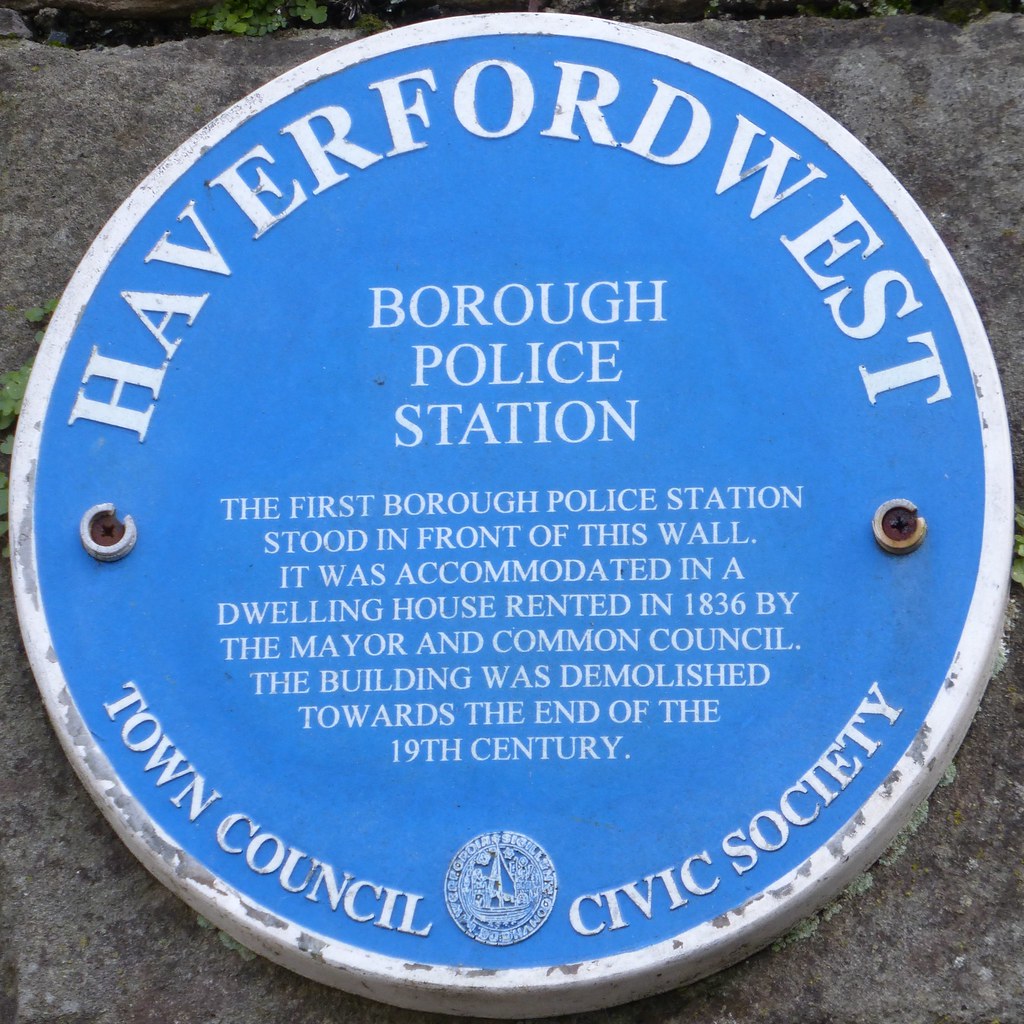The image is a detailed photograph of a blue, circular metal plaque with a white border, mounted on a gray stone wall. The plaque prominently reads "Haverford West" at the top in large white letters. Below, in smaller white text, it states "Borough Police Station." Further down, it provides historical information: "The first Borough Police Station stood in front of this wall. It was accommodated in a dwelling house rented in 1836 by the Mayor and Common Council. The building was demolished towards the end of the 19th century." At the bottom of the plaque, the text reads "Town Council Civic Society," flanking a logo that appears to be a mixture of white and light blue. The plaque is secured to the wall with screws on the left and right sides. In the background, there is a gray cement wall or boulder, with a small portion of greenery peeking in at the very upper edge, indicative of some cracks in the stone.